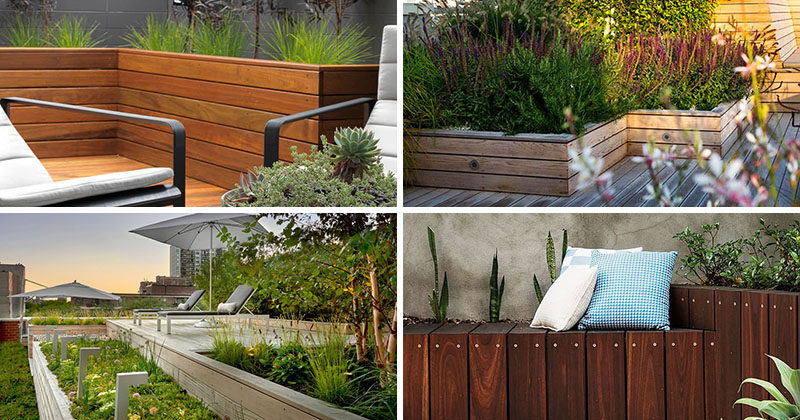This image is a detailed collage of four horizontally rectangular photos arranged in a two-by-two grid, each depicting various themed sections of a backyard or rooftop garden with extensive woodwork.

In the upper left photo, there's a raised garden bed bordered by wooden half walls with lush green plants growing inside. The upper right photo features a knee-high, lighter wood raised flower bed filled with blooming purple flowers, also positioned on the edge of a deck. The bottom left photo captures a multi-tiered city rooftop garden, showcasing wooden decks at different levels, each accented with greenery, trees, and outdoor seating arrangements, including gray chairs with umbrellas. Lastly, the bottom right photo is a close-up of a dark mahogany wooden bench adorned with blue and white pillows, with small plants growing behind it in a slightly elevated garden bed.

Each section highlights different aspects and details of wooden structures, from raised beds to seating areas, enriching the overall landscaping with both functional and aesthetic elements.